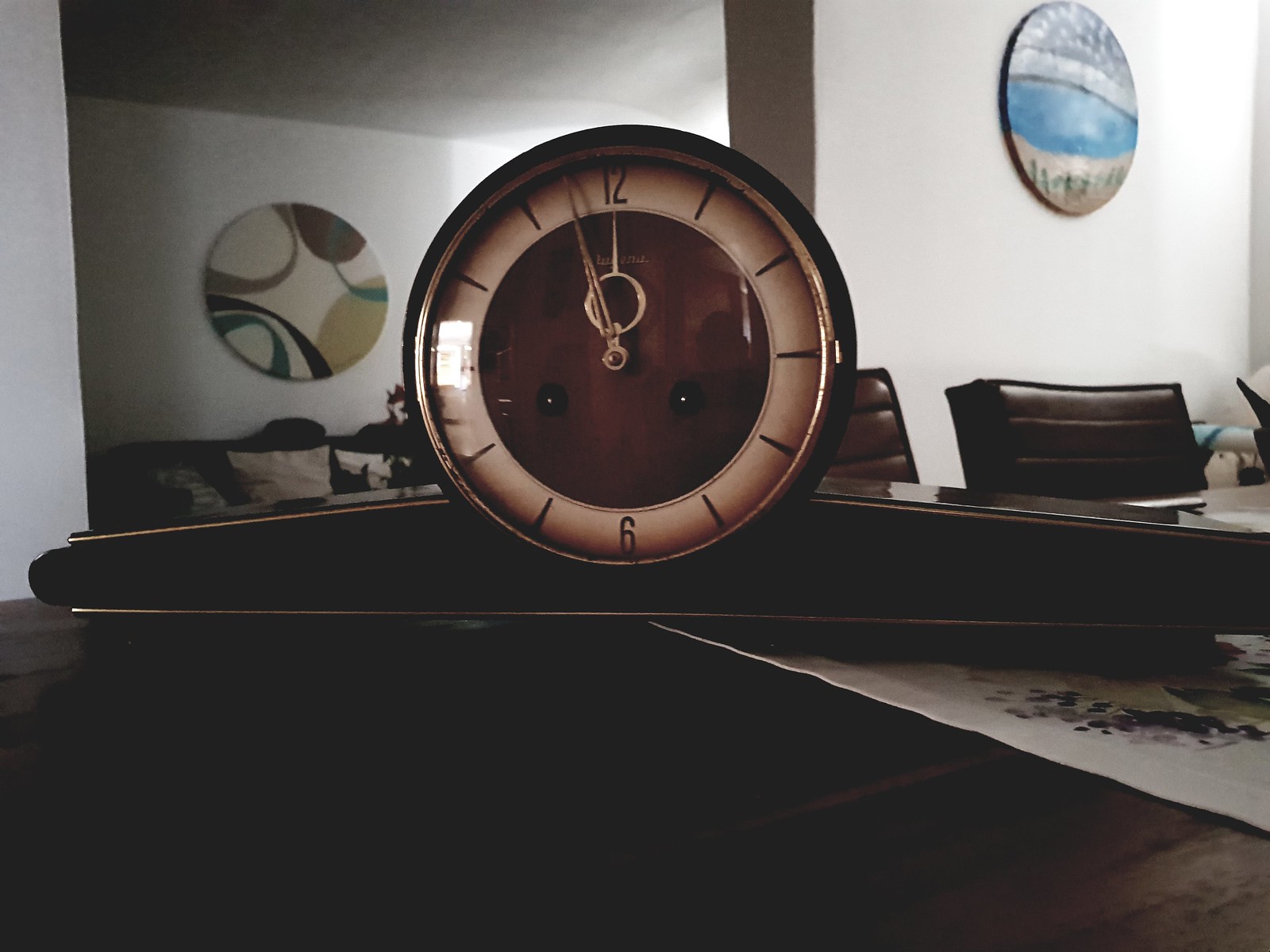The image appears to be the interior of a home, potentially serving as a dining room or office space. The photograph is centered on a dark wood dining table or desk. Prominently placed in the middle is a sleek, black, shiny object that appears to serve as the base for an antique clock perched on top. The clock is an elegant piece, showcasing a brown, old-fashioned design with gold dials, exuding a vintage charm.

Two impressive, comfortable-looking brown chairs are positioned against white walls, contributing to the room's cozy and inviting atmosphere. The walls are adorned with circular decorations. One of them seems to feature a beach scene framed within a circular motif, while another circular decoration presents an abstract design in shades of blue, brown, and black, adding artistic flair to the serene setting.